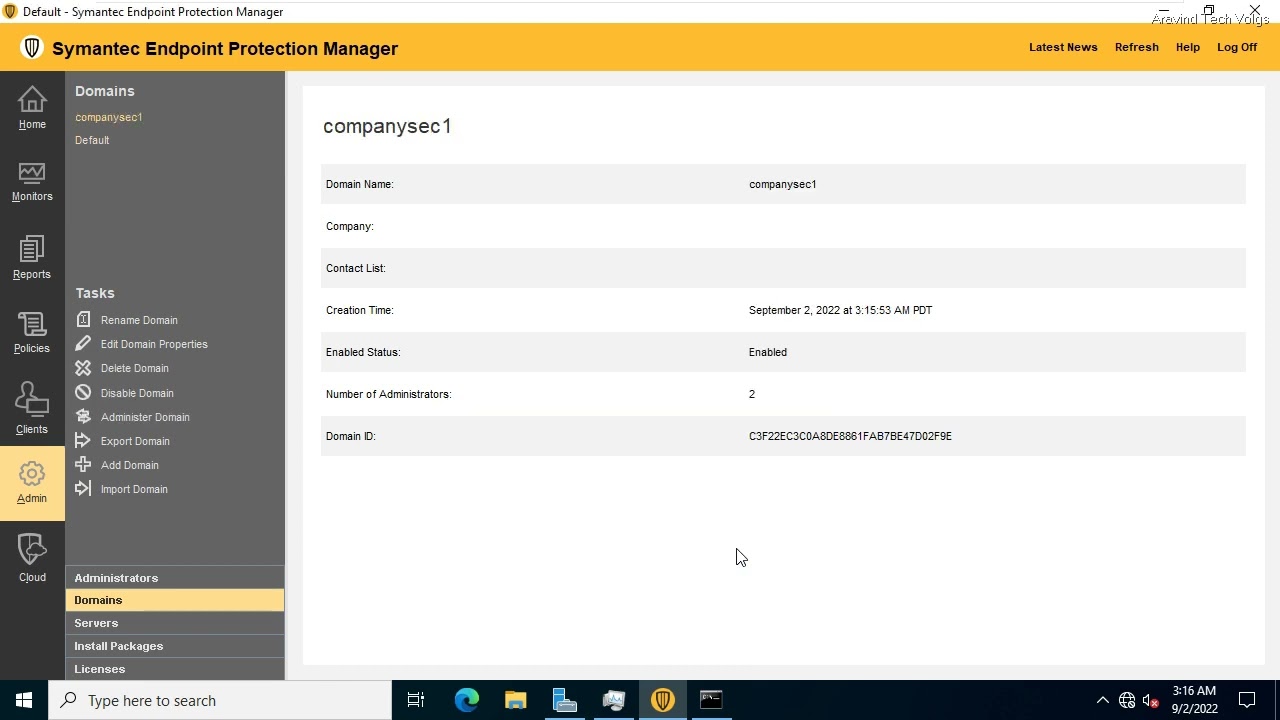This screen capture depicts the Symantec Endpoint Protection Manager interface on a computer monitor. In the top left corner, the Symantec logo is visible along with the title "Default Symantec Endpoint Protection Manager." The mustard yellow bar across the top prominently features the Symantec logo again, and the term "Symantec Endpoint Protection Manager" is printed in black lettering on the left side of the bar. To the right, options for "Latest News," "Refresh," "Help," and "Log Off" are displayed.

Beneath this top bar, the main section is divided into multiple areas. On the right, a white window showcases numerous labels that present detailed information including "Domain Name," "Company," "Contact List," "Create Time," "Enabled Status," "Number of Administrators," and "Domain ID." 

To the left of the white window, a vertical gray area serves as a navigation panel, comprising subsections accessible within the application. This gray navigation pane contains white labels including "Task," "Rename Domain," "Edit Domain Properties," "Delete Domain," "Disable Domain," "Administer Domain," "Export Domain," "Add Domain," and "Import Domain." Below these tasks are additional sections such as "Administrators," "Domains," "Servers," "Install Packages," and "Licenses."

On the far left, a thinner vertical bar in black and yellow features top-to-bottom navigation options labeled "Home," "Monitors," "Reports," "Policies," "Clients," "Admin," and "Cloud."

The active window currently displays details pertaining to "Company Section 1."

At the bottom left corner of the screen, the typical Windows interface is apparent, featuring a four-pane Start button with an adjacent search bar. The taskbar at the bottom includes usual Windows icons for the Edge Browser, File Explorer, an open program, and a Terminal window, among others. The lower right-hand corner shows the date and time in white text, indicating "3:16 AM on 9-2-2022."